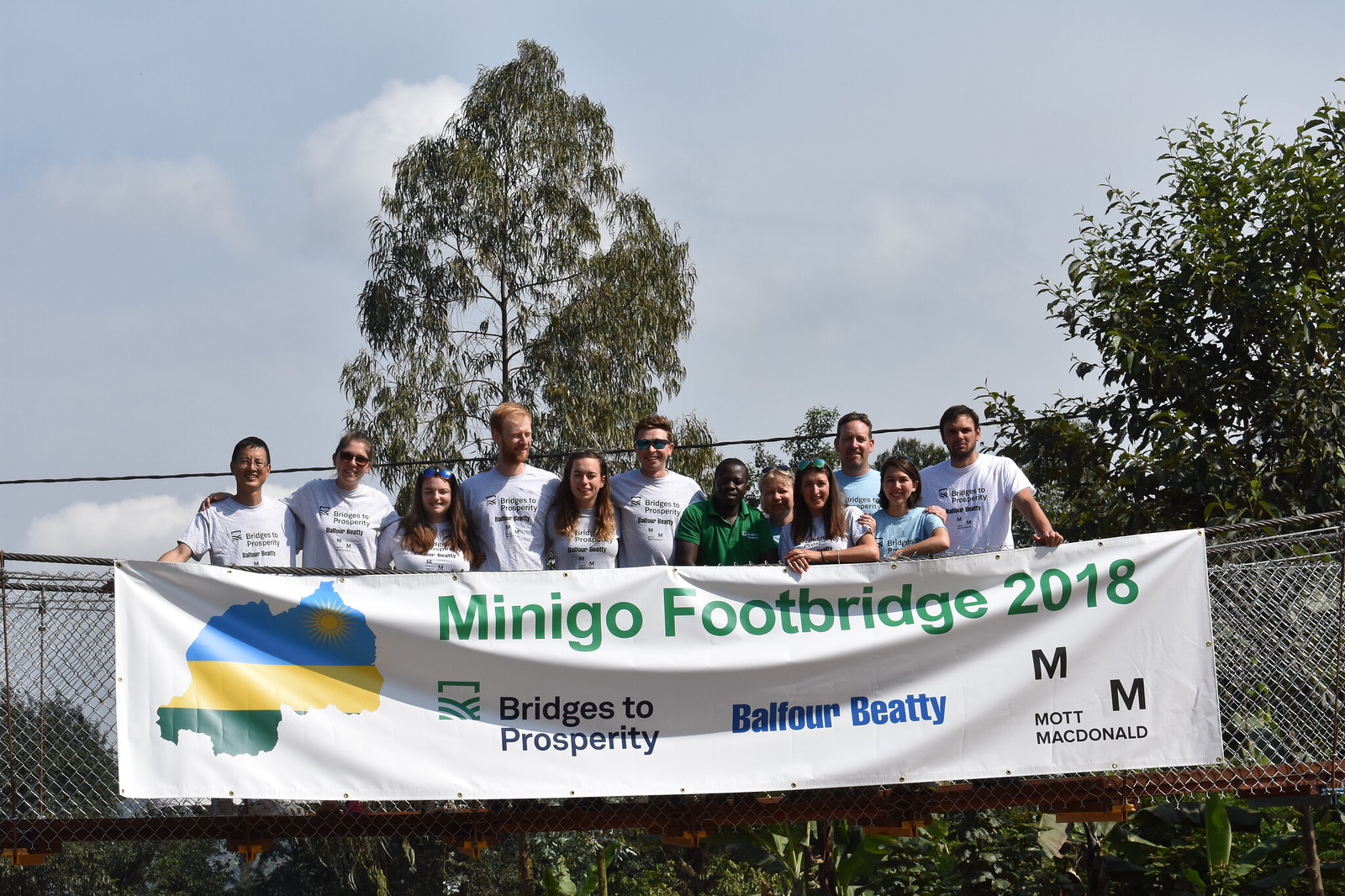This wide rectangular photograph captures a diverse group of people standing side by side on a bridge, with a prominent white banner draped over a gray metal gate in front of them. The bridge, starting from the bottom left corner and extending diagonally, features a wooden platform and white mesh sides, giving it a see-through appearance. The scene is set against a backdrop of lush green trees and a light blue sky dotted with white clouds.

Most of the people in the group, a mix of men and women likely in their younger years but not children, are wearing gray t-shirts. Notably, to the right of the first six people, a black man stands out in a green t-shirt, with five more individuals to his right. The banner they are holding reads "Minnego Footbridge 2018" in bold green letters. The left side of the banner features an image of a country in blue, yellow, and green, accompanied by the text "Bridges to Prosperity, Balfour Beatty." Towards the bottom right, two black M's are visible, followed by the words "Mac McDonald." The setting suggests a communal or team-building event focused on infrastructure and charitable work.